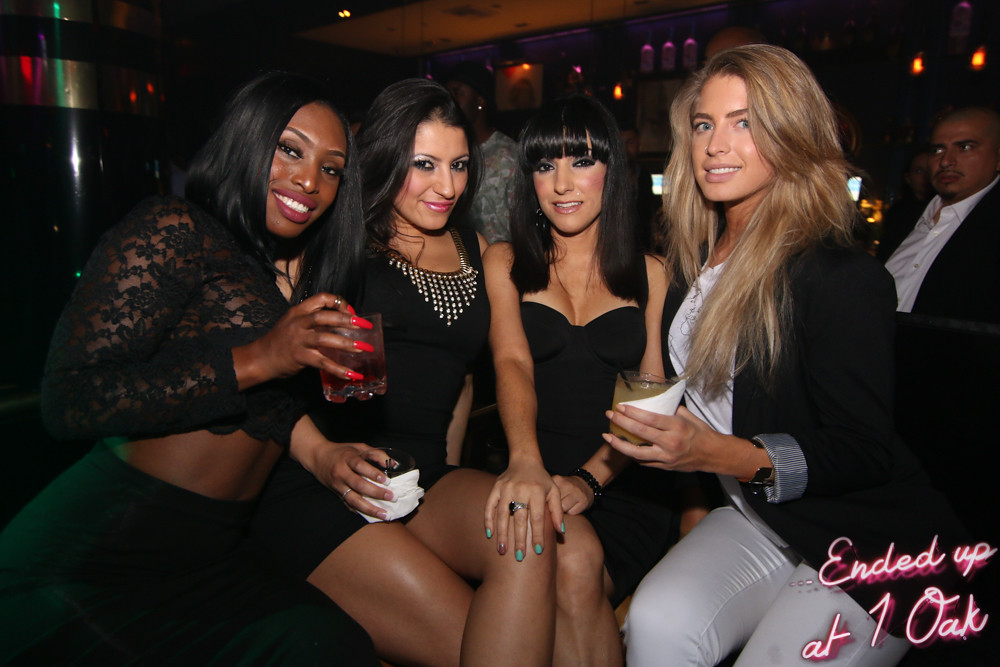This image features four women, all looking directly at the camera as they sit in front of what appears to be a bar. The background is very dark, illuminated only by a few scattered lights. 

- On the far left, a woman with black hair is dressed in a black lace top that reveals her midriff and a matching black bottom.
- Next to her, a woman with dark hair adorned with silver eye shadow is wearing a form-fitting black bodycon dress embellished with gold beads.
- The third woman, also with dark hair and bangs, is dressed in a black dress with a bustier-style top. Her bright teal-painted nails stand out vividly.
- On the far right, a dark blonde-haired woman is wearing white pants, a white shirt, and a black blazer.

In the bottom right corner of the image, "ended up at 1 OAK" is written in pink neon lettering.